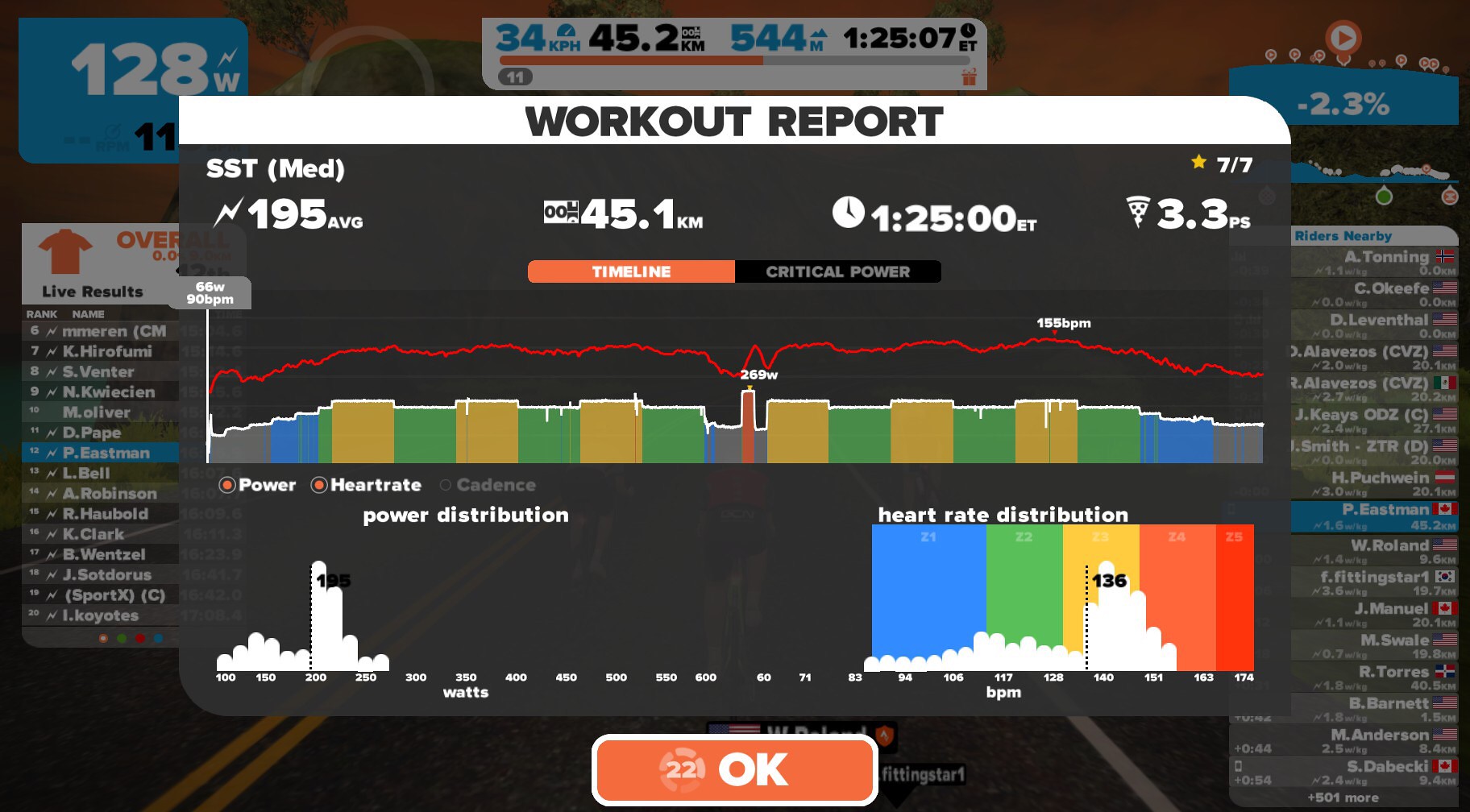The image is a detailed screenshot of a workout app displaying a comprehensive Workout Report. The central dialog box, titled "Workout Report," overlays a background that includes additional statistics, like "Riders Nearby" on the right side. Within the dialog box, key data points are displayed: the user exercised for 1 hour and 25 minutes (ET), covering a distance of 45.1 kilometers. Their average heart rate was 195 BPM, and they burned enough calories equivalent to 3.3 slices of pizza (PS, represented by a pizza icon). Beneath these metrics, there is a timeline graph that traces the user's power output and heart rate throughout the workout. Further, two bar graphs provide additional insights: one illustrating power distribution with watts on the x-axis, and the other showing heart rate distribution with BPM on the x-axis. These bar graphs feature various colors—blue, green, gold, and purple—with no legend to clarify their meanings. At the bottom of the dialog box, a large red "OK" button is prominently displayed. The surrounding elements and additional data emphasize that this app not only tracks personal fitness metrics but also allows users to compare their performance with friends.